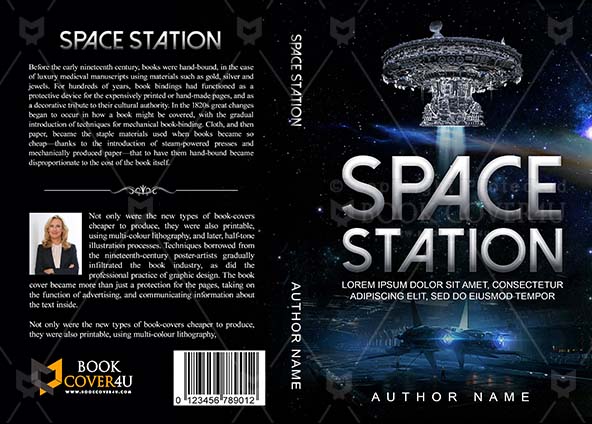This image displays an unfolded book cover for "Space Station," with a black background and grayscale details. The front cover, positioned on the right side, showcases an artistic rendering of a satellite in gray, white, and black hues, captioned "Space Station" in bold white letters. Below the title is placeholder text "Lorem ipsum dolor sit amet," indicative of text yet to be finalized. At the bottom, "author name" is inscribed in white. The spine, centrally located, repeats the title "Space Station" and "author name." The back cover, on the left side, also bears the title "Space Station" and features two sections of placeholder text. The upper segment discusses historical bookbinding, although it's partially obscured. The lower portion includes a segment about lithographic printing. Accompanying this text is a photograph of a blonde woman in a black jacket and white blouse, smiling with folded arms. At the bottom of the back cover, the publisher's name "Book Cover For You" is inscribed along with a UPC code "123456789012."